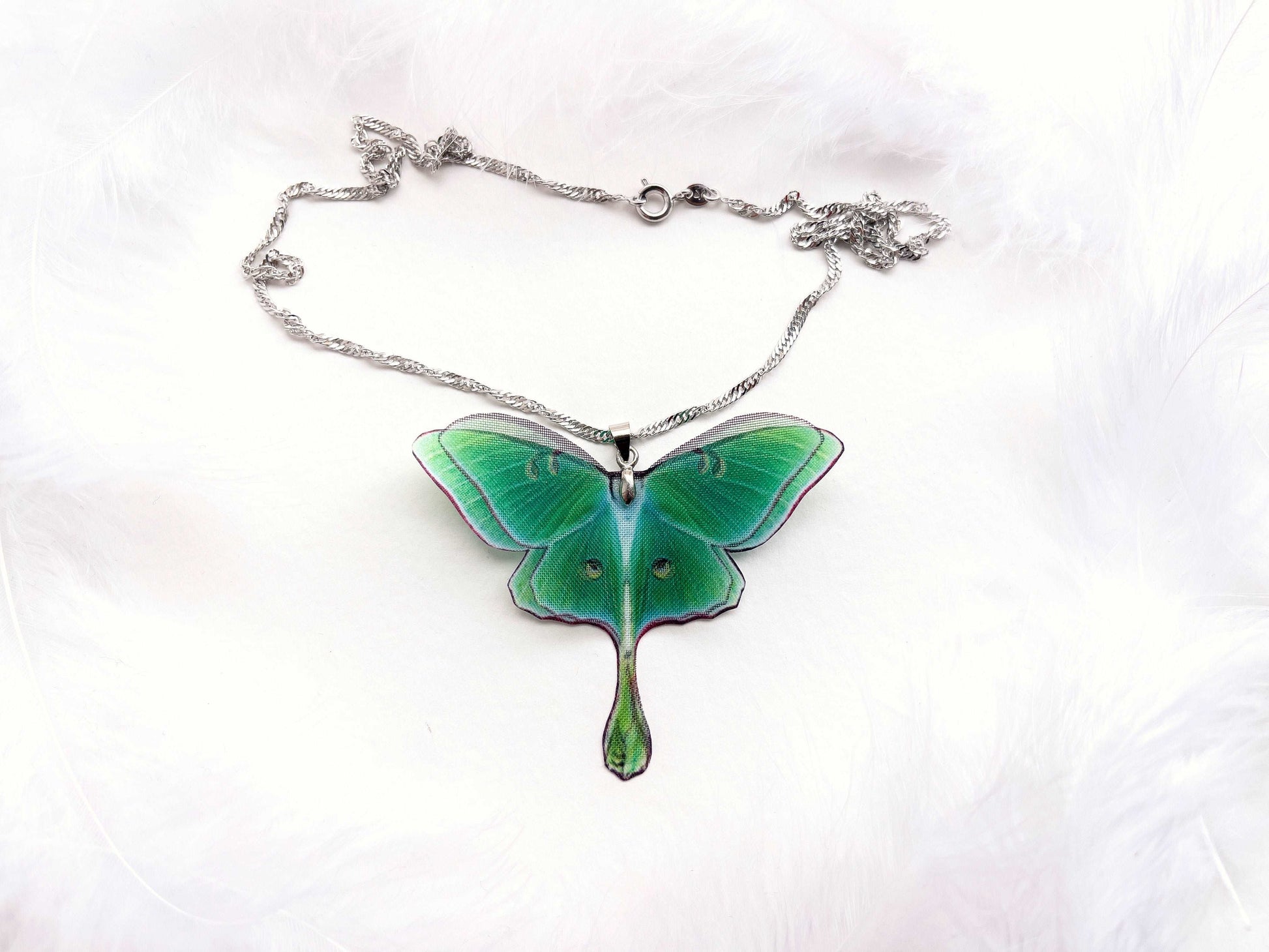This detailed photograph showcases a sterling silver strand necklace, approximately one-eighth of an inch thick, featuring a large, intricate green butterfly pendant that measures around two inches by two inches. The necklace chain, quite lengthy at an estimated 16 to 18 inches, has a spring ring clasp and is laid flat, albeit somewhat messy and knotted in the right-hand corner. The butterfly pendant, reminiscent of a Luna Moth, presents a three-dimensional, realistic appearance with sheer green hues, eye spots, and a teardrop-shaped tail. The background of the image is a whitish-gray, airy marbled surface, providing a soft, elegant contrast to the vivid, detailed pendant. The entire setup appears meticulously composed, blending photorealistic elements with possible artistic enhancements.